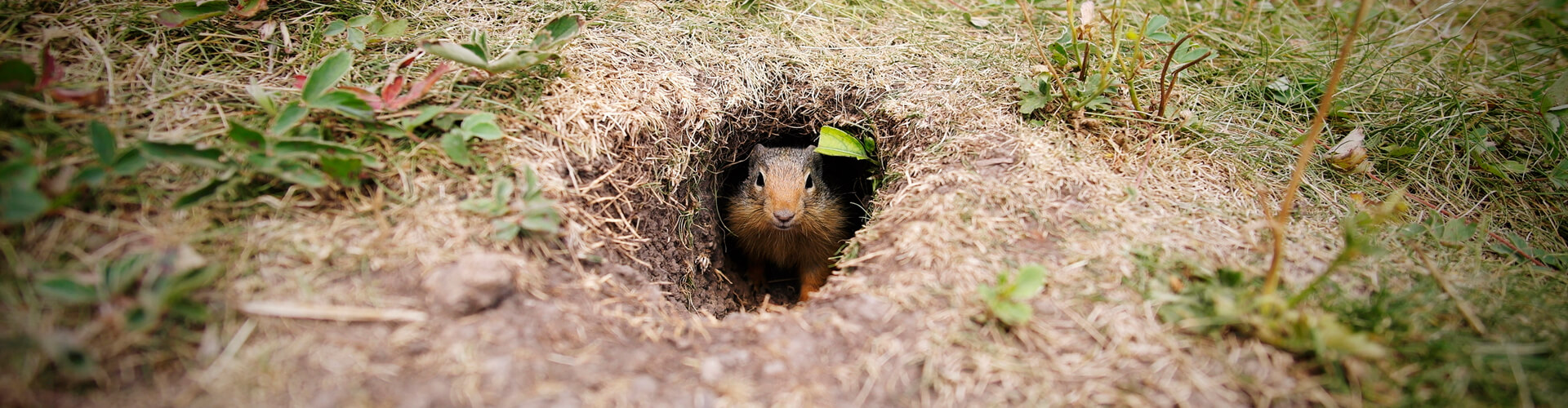In this detailed picture, we observe an outdoor setting featuring a burrowing animal, possibly a groundhog, gopher, or squirrel, nestled in its underground hole. The setting appears to be a dry forest environment with sparse vegetation primarily comprised of brown dried grass, dirt, twigs, and some greenery, including a few green and red leaves. The animal, brown in color, is seen peeking out of its burrow with a green leaf partially over its head. The shot, taken from a straight-on perspective, captures the little creature's face and part of its arm as it gazes directly into the camera. The image displays a palette of browns, greens, beiges, and a hint of pink, highlighting the rustic and natural ambiance around the burrow.